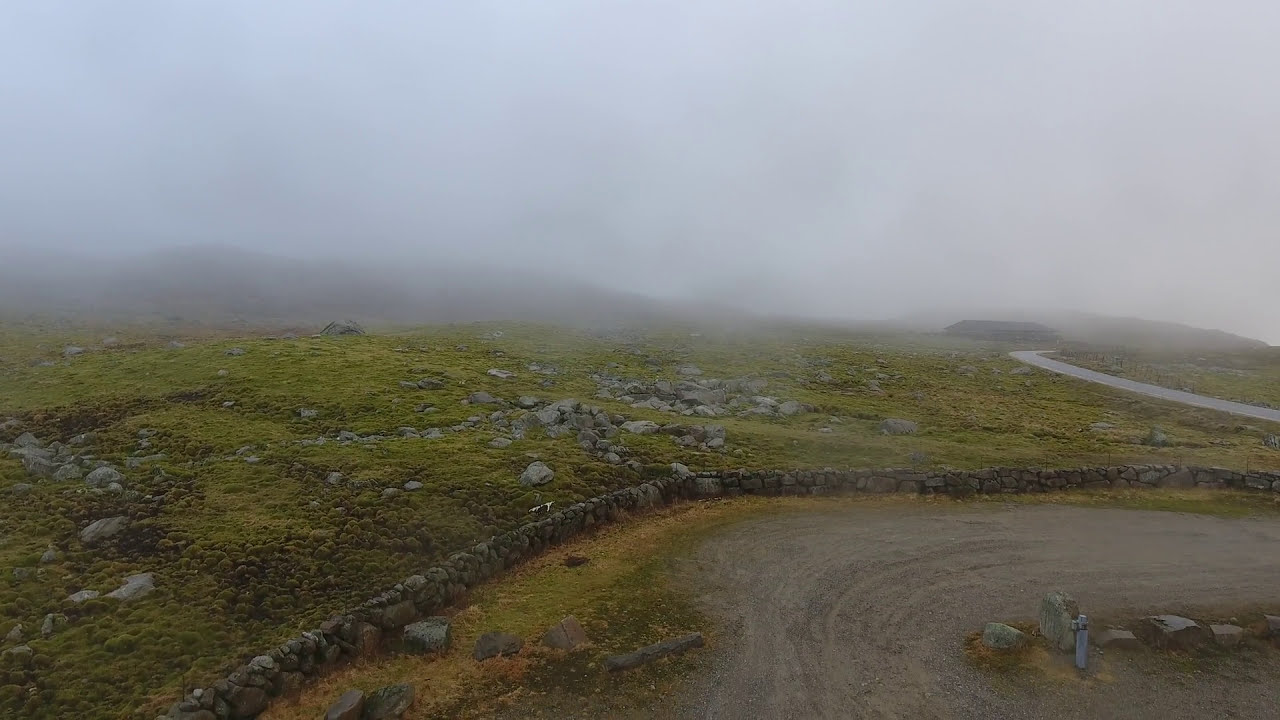The image portrays a gravel road that curves off to the right, bordered by a low stone wall. This road appears wider than a typical path and seems to be a small pull-out or parking area next to a grassy, rocky terrain. The ground cover is predominantly green, dotted with gray rocks and small vegetation, resembling moorland. In the foreground, on the bottom right, there are some scattered rocks within the gravel area. As the road curves into the distance, it disappears into a thick fog or mist that envelopes the upper half of the image, obscuring the sky and distant landscape. On the hillside behind the stone wall, the area is strewn with more gray stones and greenery. A small, low building or shack is visible in the center right, partially shrouded by the fog. The scene suggests a foggy, remote landscape, possibly reminiscent of a rural or countryside area known for its misty conditions.